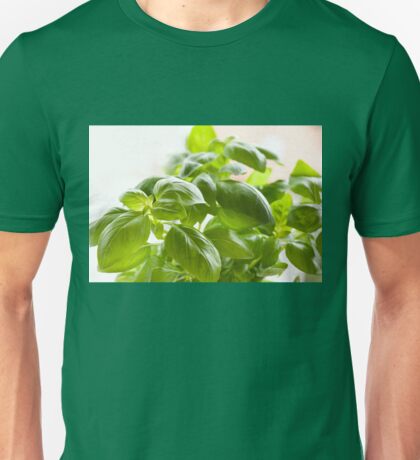The image showcases a man from the neck down wearing a dark green or forest green, short-sleeved, crew-neck cotton t-shirt. Prominently displayed on the chest area is a large, square graphic with a white background, featuring a plant with an array of green leaves in varying shades, suggestive of some sunlight giving a slight glare at the top. The man's arm muscles are visible and appear fairly toned. The t-shirt is smooth, with few wrinkles, emphasizing its cotton material. The vertical rectangular photograph captures the man’s torso, focusing on the intricate details of the shirt and its botanical design, while excluding his head and ending at his waist.